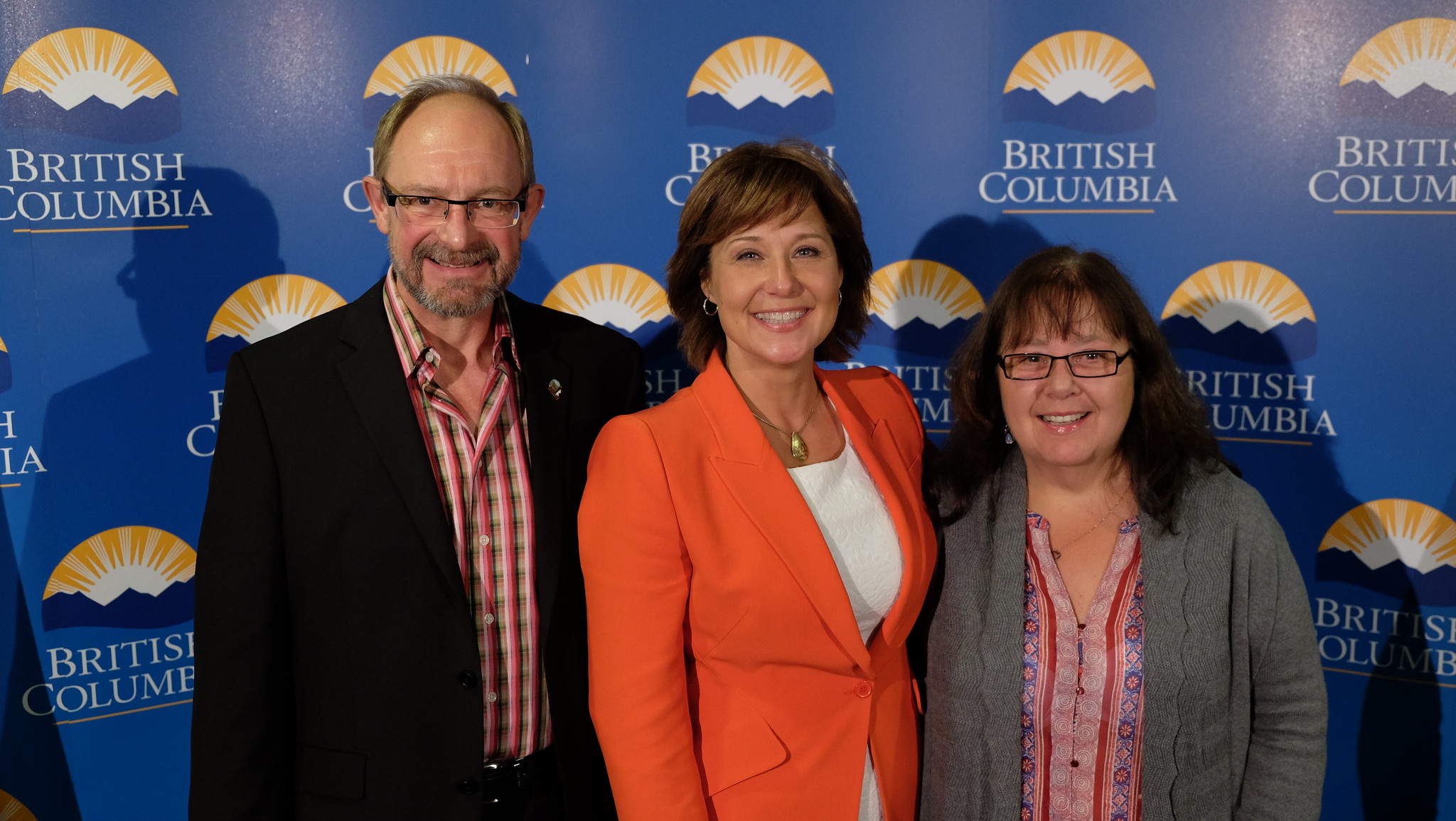In this image, three individuals are posing for a photograph against a dark blue backdrop adorned with a repeating logo that features a mountain with a sunburst and the words "British Columbia" in white text. The people are standing in the center of the image, looking directly at the camera and smiling. 

On the left is a man dressed in a black business coat, a brown, red, and white checkered button-up collared shirt, black pants with a black belt and a silver buckle, and black-framed glasses. In the middle stands a woman with short brown hair, wearing an orange business coat over a white blouse, accessorized with a gold necklace with a gold pendant and silver hoop earrings. To the right is another woman with longer brown hair and glasses, dressed in a gray sweater coat and a pink and red floral-patterned top. The setting appears to be indoors, potentially during a company meeting or event. The vibrant colors of their attire contrast with the dark blue backdrop, creating a striking and professional portrait.